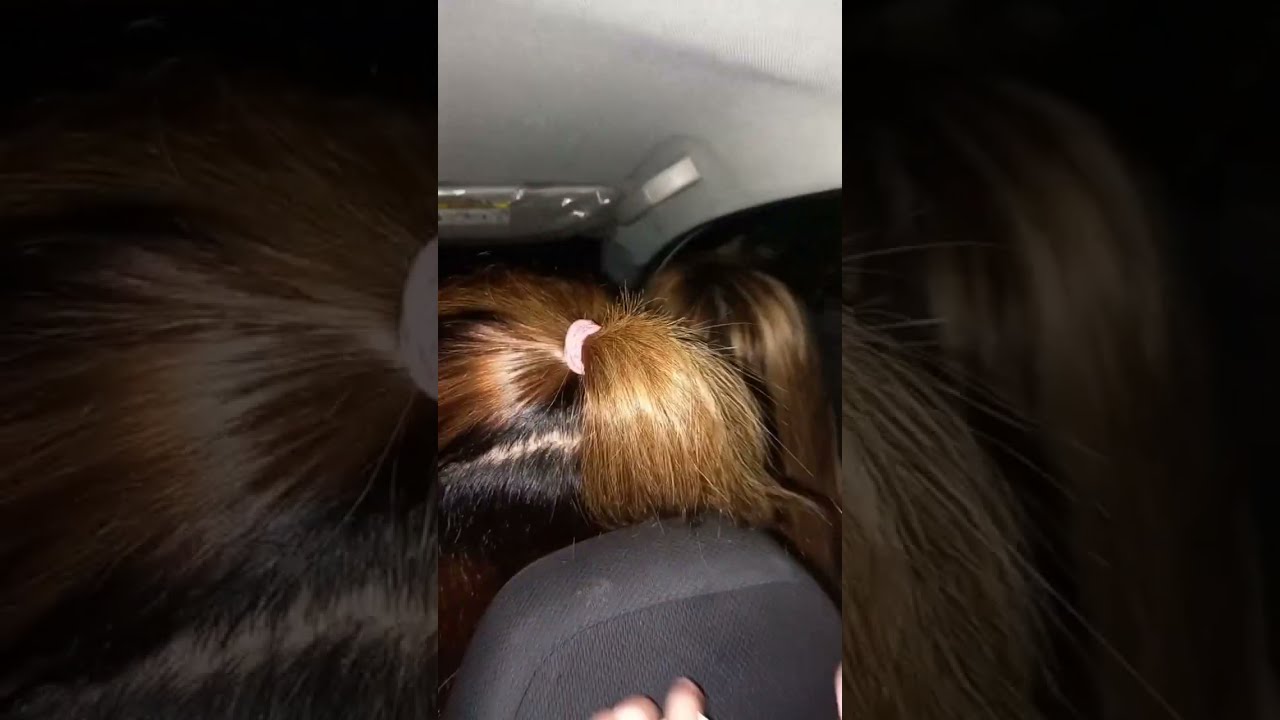The photograph captures the back interior of a vehicle at night, taken vertically with a cell phone. The central focus is the back of the front passenger seat, showing the back of a person's head. This individual has hair tied into a ponytail with a light-colored (pink) scrunchie. Their hair is dark at the roots, transitioning to a lighter brown towards the ponytail, making it difficult to determine their gender. Just visible to the right is another person with long brown hair, likely also sitting in the front seat. The background shows the dark outside through the vehicle's window, suggesting a nighttime setting. The interior of the car is illuminated by a light source from behind the camera, revealing part of the passenger side window, a strip of the windshield, a small handle bar on the car roof, and a sun visor. The photographer’s hand rests on the seat cushion of the front passenger, contributing to the intimate, candid nature of the image.